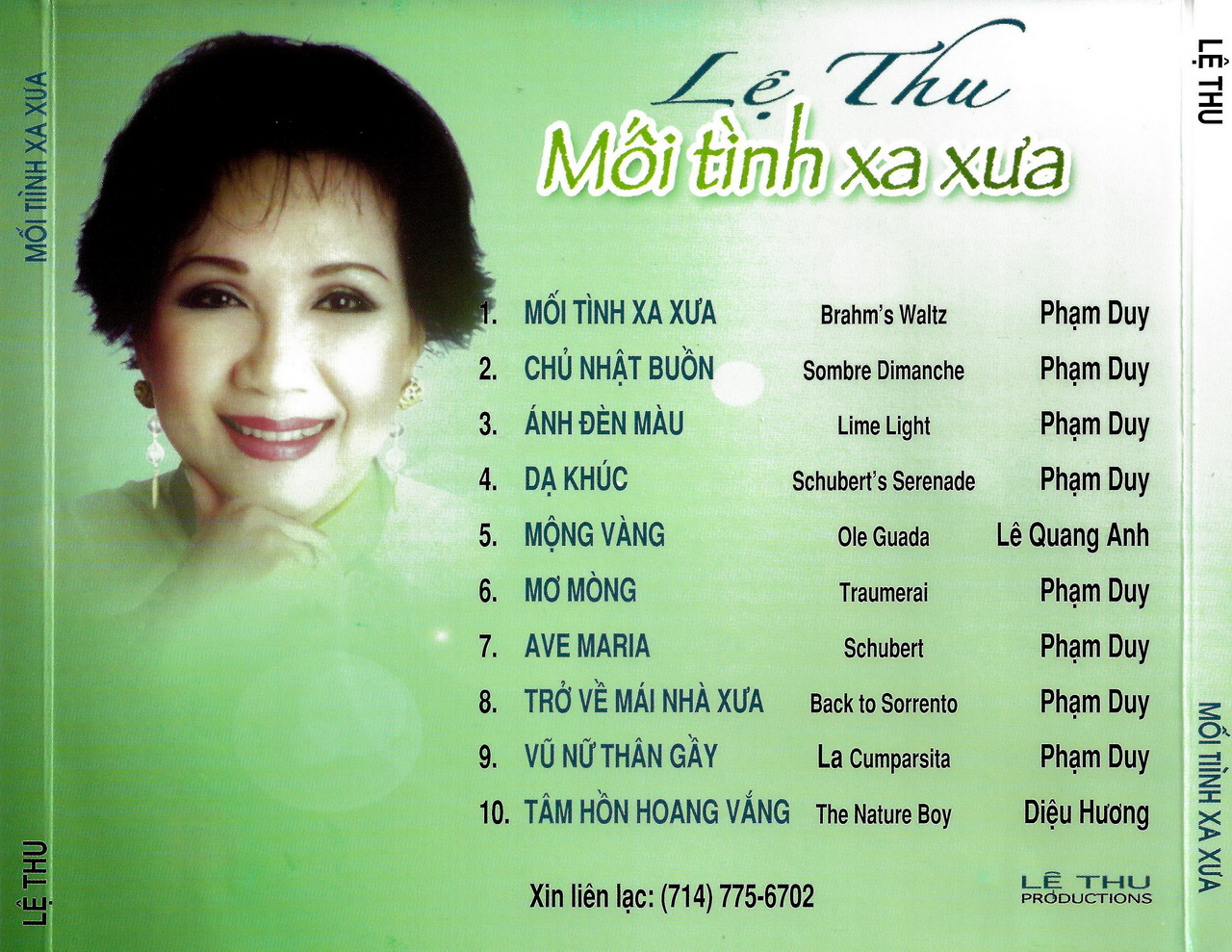The image showcases the back cover of a CD with a predominantly green background, transitioning to white in the upper right corner. Prominently displayed in blue text at the top right is the name "Lê Thu," followed by "Moy Tinh Xua," likely the title of the album, in green and white text. A list of ten Vietnamese song titles, featured in the center of the cover, includes "Brahms Waltz," "Sombra de Manache," "Limelight," "Schubert Serenade," "Ali Guada," and "Nature Boy."

In the upper left of the cover, there is a photograph of a Vietnamese woman. She has short brown hair, wears drooping earrings and makeup, including lipstick, and is smiling. Her hand rests gently under her chin, though the image fades below her hand. Her name, assumed to be Lê Thu, suggests she may be the artist of the album. The right column mentions Pham Duy, possibly indicating the author or contributor of the music.